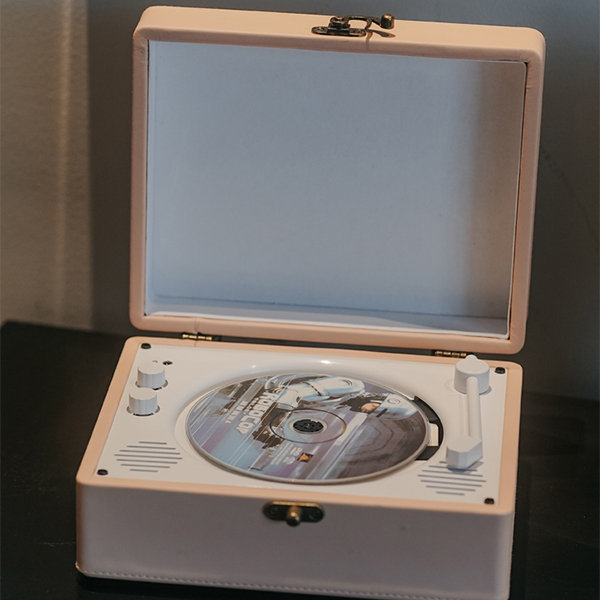The image depicts a vintage-style record player housed in a pink carrying case with burnished gold hardware. The white box-like player is open, displaying a CD with "Robocop" written on it, featuring an image of a robotic figure. The player's lid is held by two hinges, and there’s a latch for securing it when closed. To the left of the CD slot are two white knobs, likely for volume control, while on the right, there is a white arm that is presumably used to play records. The record player also features speaker lines on each of the lower corners. The device is positioned on a dark-colored table against a grey background, which appears to be a curtain.